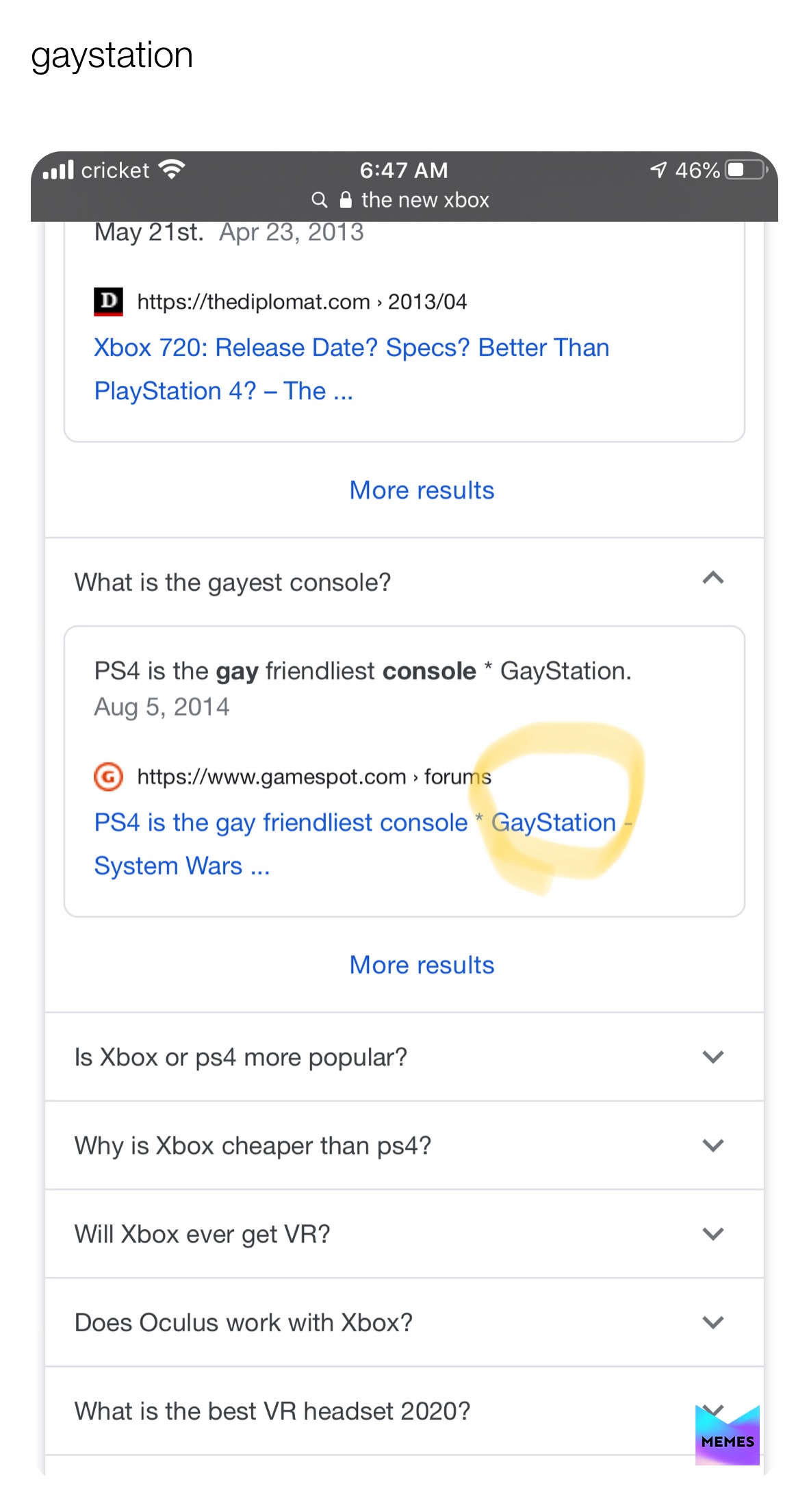Taken from a cell phone screen, this image showcases various interface elements and content. In the upper left corner, within a gray banner, there are four bars indicating wireless signal strength next to the word "Cricut," along with the time "6:47 AM." Adjacent to these is a search icon with a lock symbol, labeled "the new Xbox."

In the upper right corner, there is an arrow pointing upward and to the right, accompanied by "46%" and a battery icon displaying a nearly half-full charge. Below this, in white text on a gray box, the dates "May 21st, April 23rd, 2013" are shown alongside a link to an article from thediplomat.com titled "Xbox 720 Release Date Specs Better than PlayStation 4."

Further down, there is a blue row labeled "more results." Beneath it, a highlighted question appears: "What is the gayest console?" This is followed by a box stating that the "PS4 is the gayest, friendliest console," referred to as "Gay Station" from August 5th, 2014. A "G" circle logo is visible, linking to forums on www.gamespot.com, reiterating the label "PS4 is the gay-friendliest console" with "Gay Station" highlighted in yellow.

Additional results and queries follow, asking "Is Xbox or PS4 more popular?" and "Will Xbox ever get VR?" Near the bottom right corner, a blue-purple "M"-shaped logo is visible, associated with the term "memes."

This detailed caption captures the entirety of the onscreen information visible in the image.